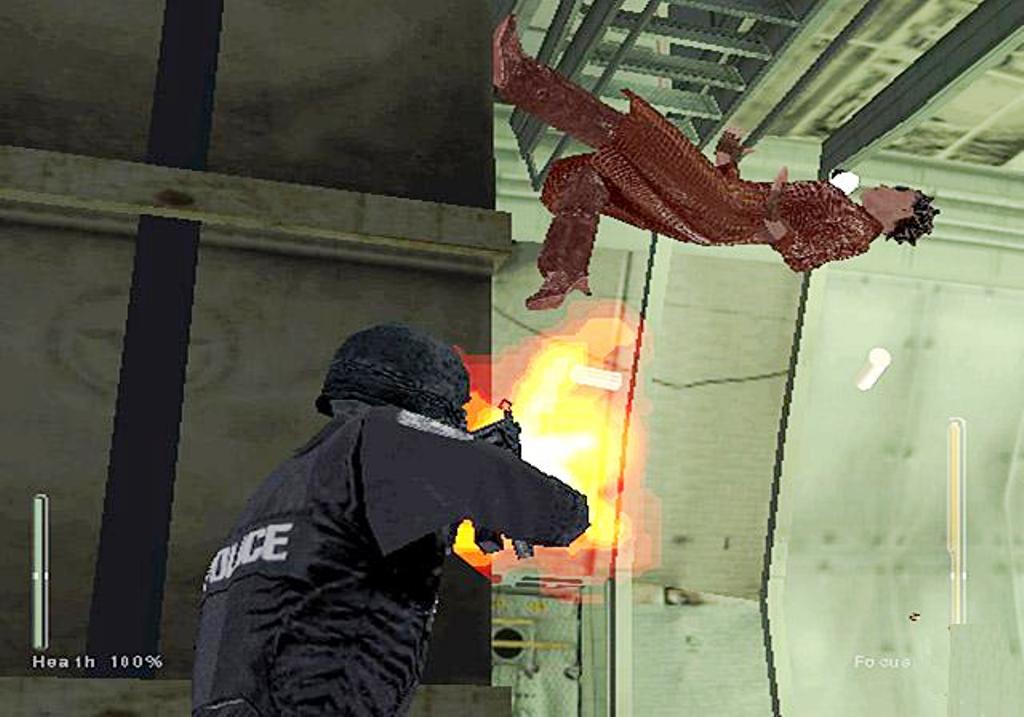This screenshot from a video game depicts a dynamic action scene set against a greenish-gray wall adorned with industrial elements such as pipes, steel bars, and a fluorescent light positioned on the lower right side. The central characters in the scene are a police officer and a person in a striking red and gold outfit.

The police officer, clad in an all-black uniform including a helmet and a bulletproof vest labeled "POLICE" on the back, is captured in the act of firing a gun. Flames can be seen bursting from the gun's muzzle, indicating a discharge. The officer's right arm is bent at the elbow, holding and aiming the gun slightly upwards and to the right. Behind the officer, additional environmental details include a vertical black pole running up the gray wall with trim and an adjacent lighter blueish-gray wall.

Running away from the officer in the image is a person—presumed to be a woman—wearing a vivid red and gold sequined outfit that includes a long coat, pants, and high-heeled shoes. She has short, spiky black hair and is depicted in mid-motion, with her left arm bent and raised at the waist and her right hand slightly lower. Her dynamic pose, with one foot on the wall and the other pointed downwards towards the officer, creates an intense sense of action and movement.

Additionally, a vertical health bar labeled "Health 100%" is prominently displayed in the lower-left corner of the screen, adding to the overall context of the video game interface.